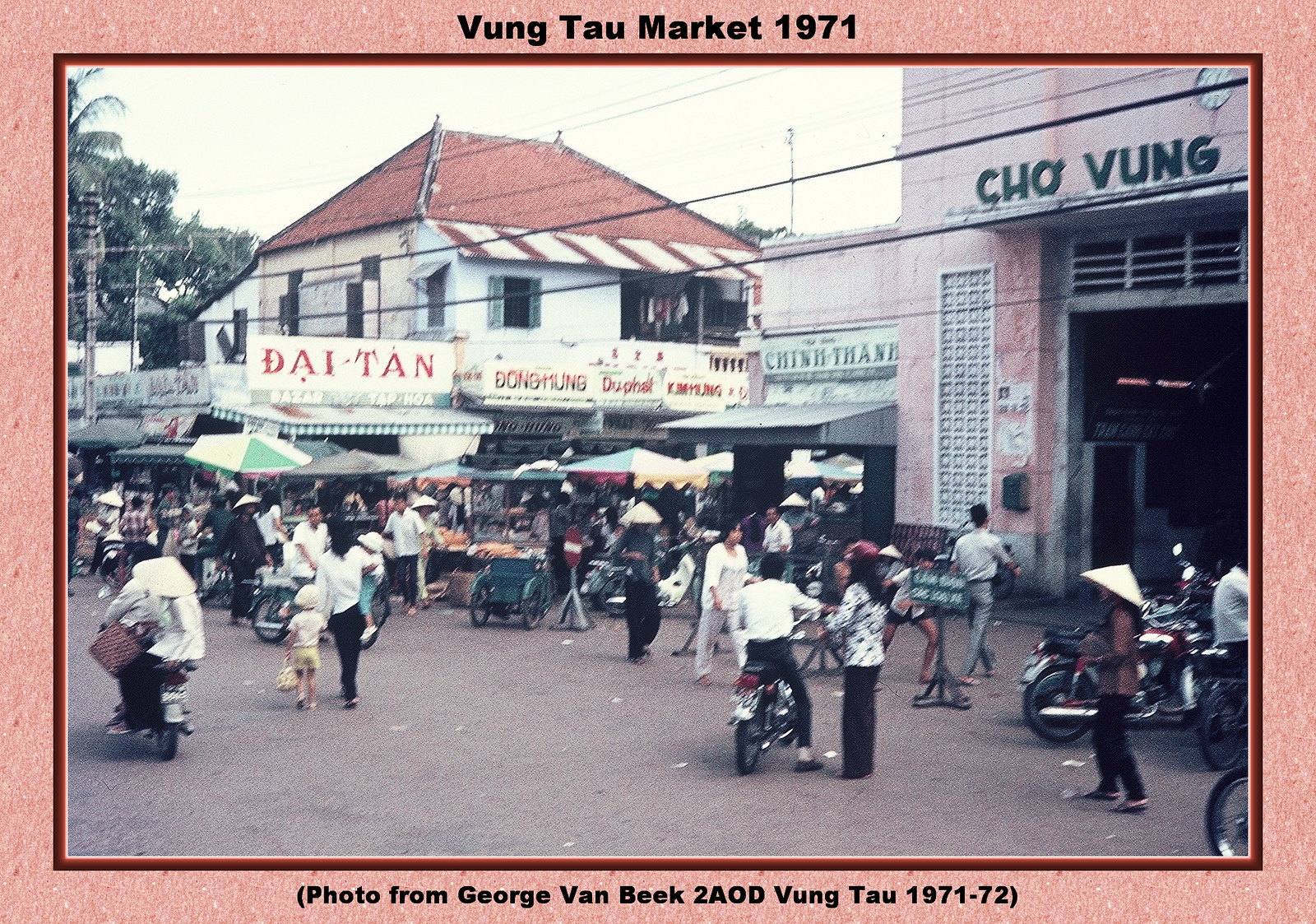The image is a color photograph capturing a bustling Vietnamese market in 1971. This outdoor market features a concrete or asphalt groundscape with various vendors and booths lining the perimeter of the open area. People are actively walking about, some riding scooters or motorcycles, while others accompany small children. Dominating the right side of the picture is a large concrete or brick building with the words "CHÔ VŨNG" displayed prominently above a sizable entrance. 

In the center, there is a red-roofed structure with open windows, leading to an area crowded with different street vendors. Among the visible shop signs are "DAI TÀN," "Dong Hung," "Kim Hung," and "Du Phat." The backdrop includes trees in the top left corner and a blue sky peeking through. 

The photograph is framed by a red border that includes text reading "VŨNG TÀU MARKET 1971" at the top and "PHOTO FROM GEORGE VAN BEEK TO AOD VŨNG TÀU 1971-72" at the bottom. The image, nearly square but slightly horizontal, is an evocative snapshot of a vibrant market scene, rich in colors such as brown, beige, green, and dark green.